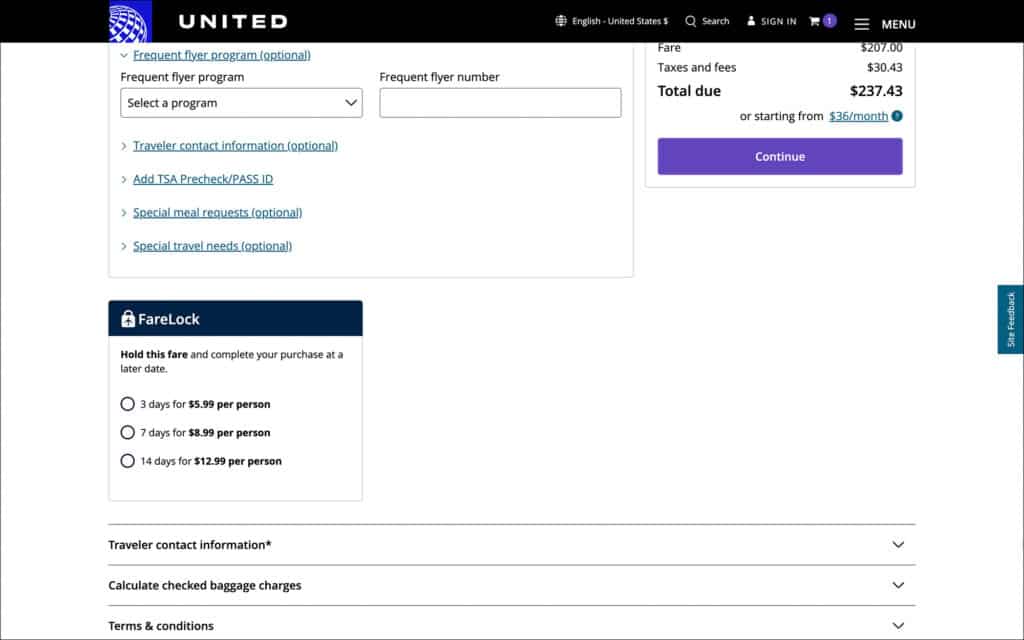This desktop screenshot from United Airlines showcases a detailed view of the checkout process nearing completion. At the upper right corner, although slightly cut off, the total fare is displayed. The fare itself amounts to $207 USD, with an additional $30.43 USD for taxes and fees, culminating in a total of $237.43 USD. The option to pay in monthly installments starting from $36 is also mentioned, indicating a payment plan. 

A prominently featured purple "Continue" button stands out on the screen. To its left, partially visible, is the section for adding a frequent flyer program and number. Below, there are additional but unselected dropdowns for optional entries such as travel contact information, TSA Pre-check/Pass ID, special meal requests, and special travel needs.

Further down, the fare lock feature is detailed, offering to hold the fare and complete the purchase later: 3 days for $5.99 per person, 7 days for $8.99 per person, and 14 days for $12.99 per person. Below this, more dropdowns appear for required traveler contact information (indicated by an asterisk), the calculation of checked baggage charges, and terms and conditions.

The interface is displayed in light mode, characterized by a white background accented with black borders and a black header.